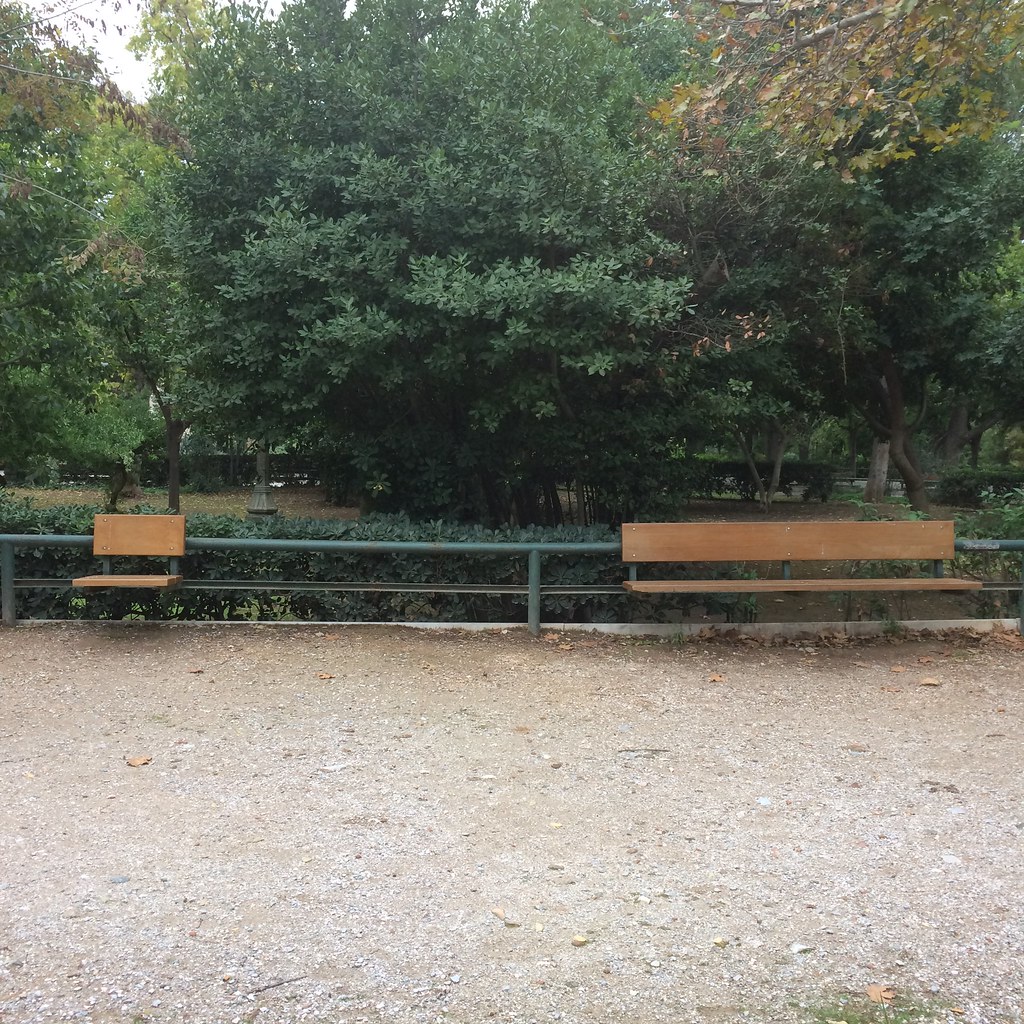The image depicts a section of a park characterized by a ground covered in dirt and small rocks, interspersed with old leaves. Among the notable features are two benches positioned against a short, green metal fence. On the left side, there is a small, brown bench designed to seat a single person. In contrast, the right side of the image showcases a much longer brown bench, which can accommodate multiple people, likely around four or five. The scene is framed by lush greenery, including numerous trees that cast varying shades of light and shadow across the area, making parts of the background harder to discern. Towards the rear of the park, partially obscured by tree shade, there appear to be statues. The overall lighting suggests it is daytime, as indicated by the glimpses of the sky visible through the trees.